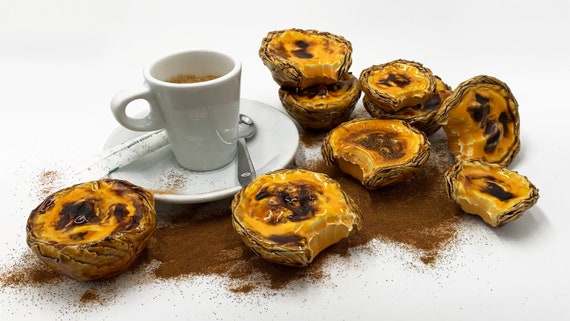The image displays a white coffee mug, about three-quarters full with a light brown liquid, assumed to be coffee, with the handle facing left. The mug rests on a white plate, accompanied by a silver spoon on its right. Surrounding the bottom and right side of the mug are nine halves of a round fruit resembling coconuts, but with orange insides and brown centers. The fruits are sprinkled with what appears to be cinnamon, which is also scattered generously on the plate. The setup is placed on a light gray surface, giving the overall image a clean and neatly arranged appearance.